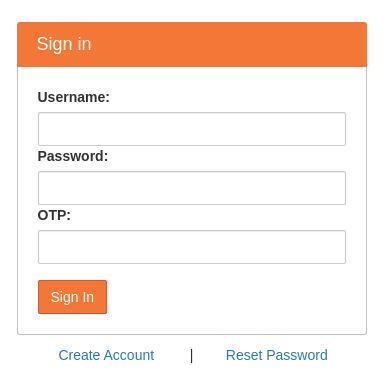### Detailed Caption:

This image is a screenshot from a sign-in page. The top portion of the image showcases a header area that is almost a perfect square, encapsulated by black lines on the left, right, and bottom edges. The top edge, however, is marked by an orange border roughly an inch thick. Positioned in the top left corner of this orange border area, the word "Sign-In" is displayed in white text.

Beneath the orange header, the background transitions to white. About an inch from the top, the word "Username" is prominently displayed in bold, black text. Directly below this label, there is a rectangular input field. This rectangle spans nearly the entire width of the page, maintaining a half-inch margin on both the left and right sides. The input field itself has a white background with a thin black border.

Following the "Username" input field, the label "Password" appears, also in bold, black text. Below this is another rectangular input field, identical in style and dimensions to the "Username" field.

Further down, the label "OTP" (One-Time Password) is presented in all capital letters, followed by another rectangular input field. To the side of these fields are two dots, although their purpose is not entirely clear.

At the bottom of the input section, an orange tab that reads "Sign-In" is located in the bottom-left corner. The base of the header section transitions to a black line, completing the containment of the input fields.

Below this black line, approximately an inch from the left edge of the page, the text "Create Account" is displayed in blue, with both the "C" and "A" capitalized. Centered beneath the black line, there is another vertical black line running up and down, about half an inch in length. On the right side of this line, the words "Reset Password" appear, also in blue, with the "R" in "Reset" and the "P" in "Password" capitalized.